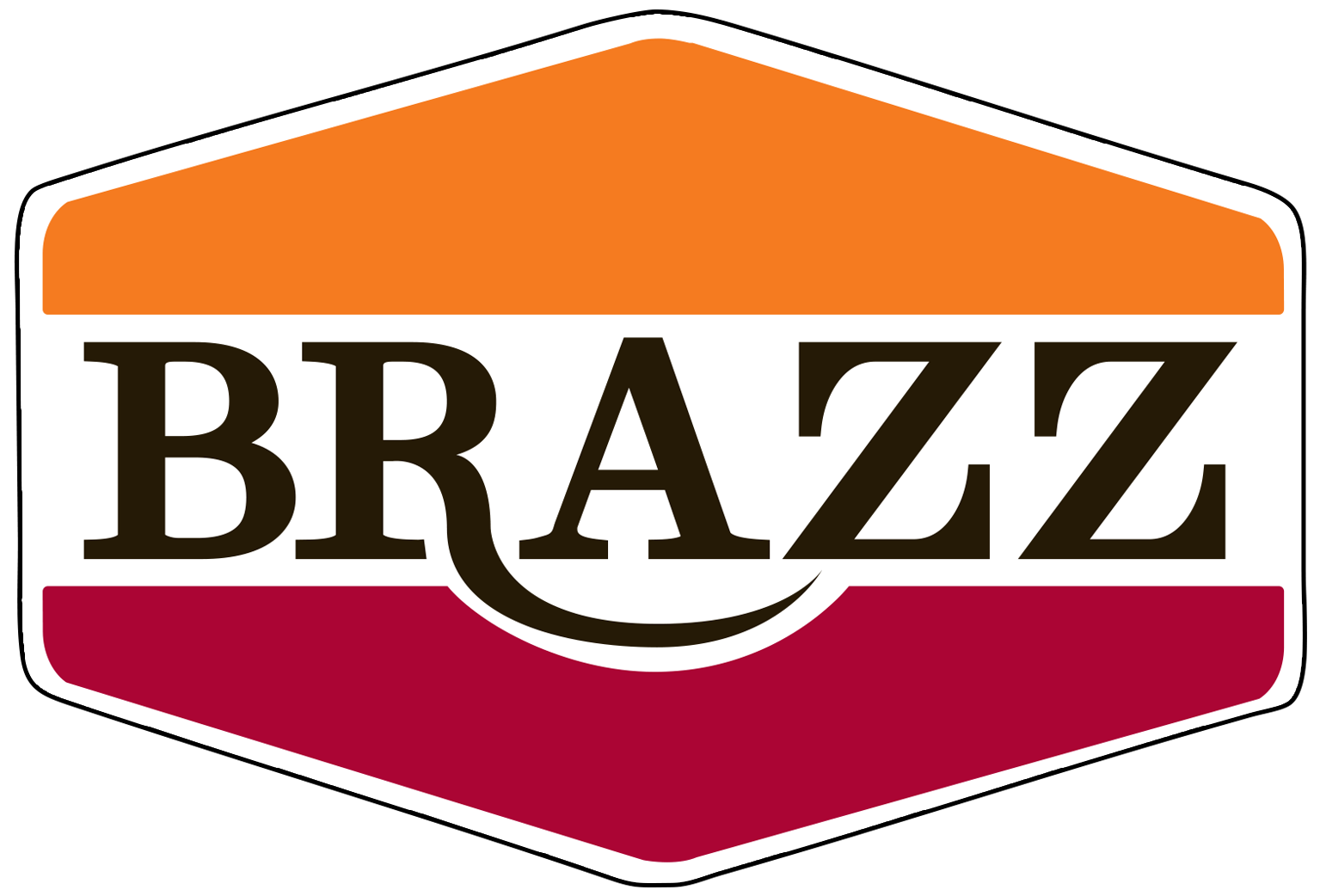The image is a logo for a company, characterized by a hexagonal shape with a thin black outline and a white background. The centerpiece of the logo is the text "BRAZZ" in bold, black letters. Notably, the tail of the "R" sweeps underneath the "A," creating a stylized curve that dips into and modifies the shape of the bottom element. Above the letters is an orange trapezoid, and a similar red trapezoid mirrors it below. The tail of the "R" cuts into the red trapezoid in a manner reminiscent of a smile, forming a distinctive divot. This detailed and balanced arrangement makes for a striking and memorable logo design.